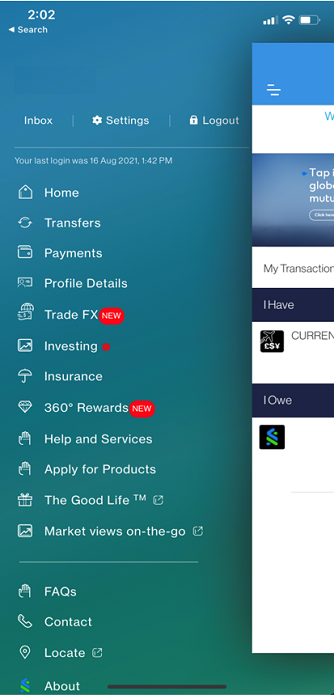Here we have a screenshot from a mobile app displayed on a mobile phone or tablet. The screenshot features an open menu on the left-hand side, causing the rest of the content to shift to the right. 

In the upper left-hand corner, the time is displayed in white as 2:02. The upper right features indicators including three of four bars for cellular data, three of three bars for Wi-Fi, and a half-full battery icon. 

The left-side menu contains several navigation options: 
1. Inbox
2. Settings
3. Logout

An account activity message states, "Your last login was August 16th, 2021 at 1:42 p.m." 

Below this are various categories, each with corresponding icons:
- Home (home icon)
- Transfers
- Payment (wallet icon)
- Profiles (person icon)
- Trade FX (dollar bill icon, marked as "NEW" in red)
- Investing (stock icon with a red dot)
- Insurance (umbrella icon)
- 360 Rewards (diamond icon, marked as "NEW")
- Help & Services
- Apply for Products (icon of a raised hand)

Additionally, there are sections for:
- Good Life TM (present icon)
- Market Views on the Go (stock icon)
- FAQs
- Contact
- Locate
- About

On the right-hand side, there is a window with a white background, partially pushed aside due to the open menu.